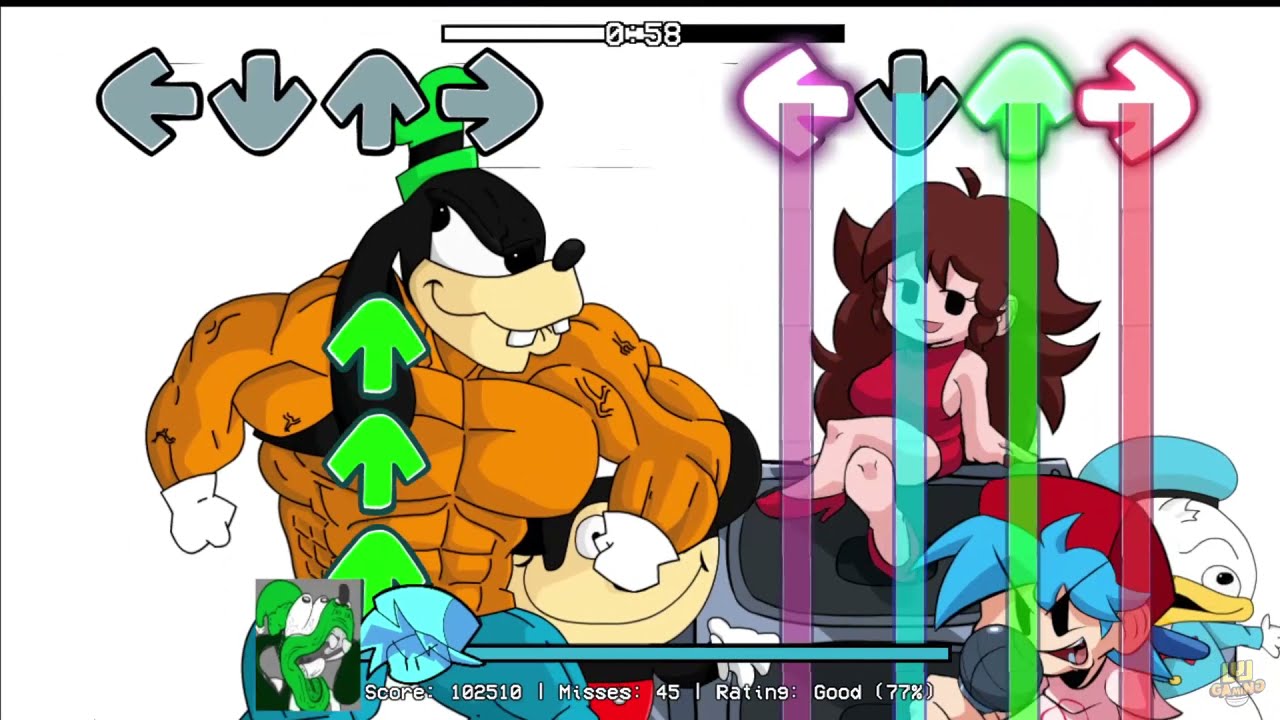The image appears to be a vibrant and chaotic scene, potentially a screenshot from a video game akin to "Dance Dance Revolution." The background is stark white, with a black line running horizontally across the top of the frame. 

On both the upper left and right corners of the image, there are sequences of directional arrows (left, down, up, right). The arrows on the left are in a grayish font, while the arrows on the right are more colorful and illuminated: purple, teal, green, and red, corresponding to vertical columns of the same colors.

Dominating the left half of the image is a stylized, muscular version of Disney's Goofy, wearing blue pants, a yellow-orange top, white gloves, and a green hat, extending almost from the bottom to the top of the image. His appearance is exaggerated with significant muscle definition.

To the right of this muscular Goofy stands a high-heeled, brown-haired woman in a red dress, resembling a potentially seductive cartoon character. Further to the right, crowded into the corner, there are more bizarre and distorted figures: a grotesque version of Donald Duck wearing a blue cap and shirt, partially obstructed by an anime-like boy with blue hair and a red hat.

Beneath these characters, there is a line of text reading "0:58," which suggests it might be the 58th frame of this game-like scenario. The entire composition hints at a whimsical yet eerie crossover of familiar cartoon characters in a surreal, game-like environment.